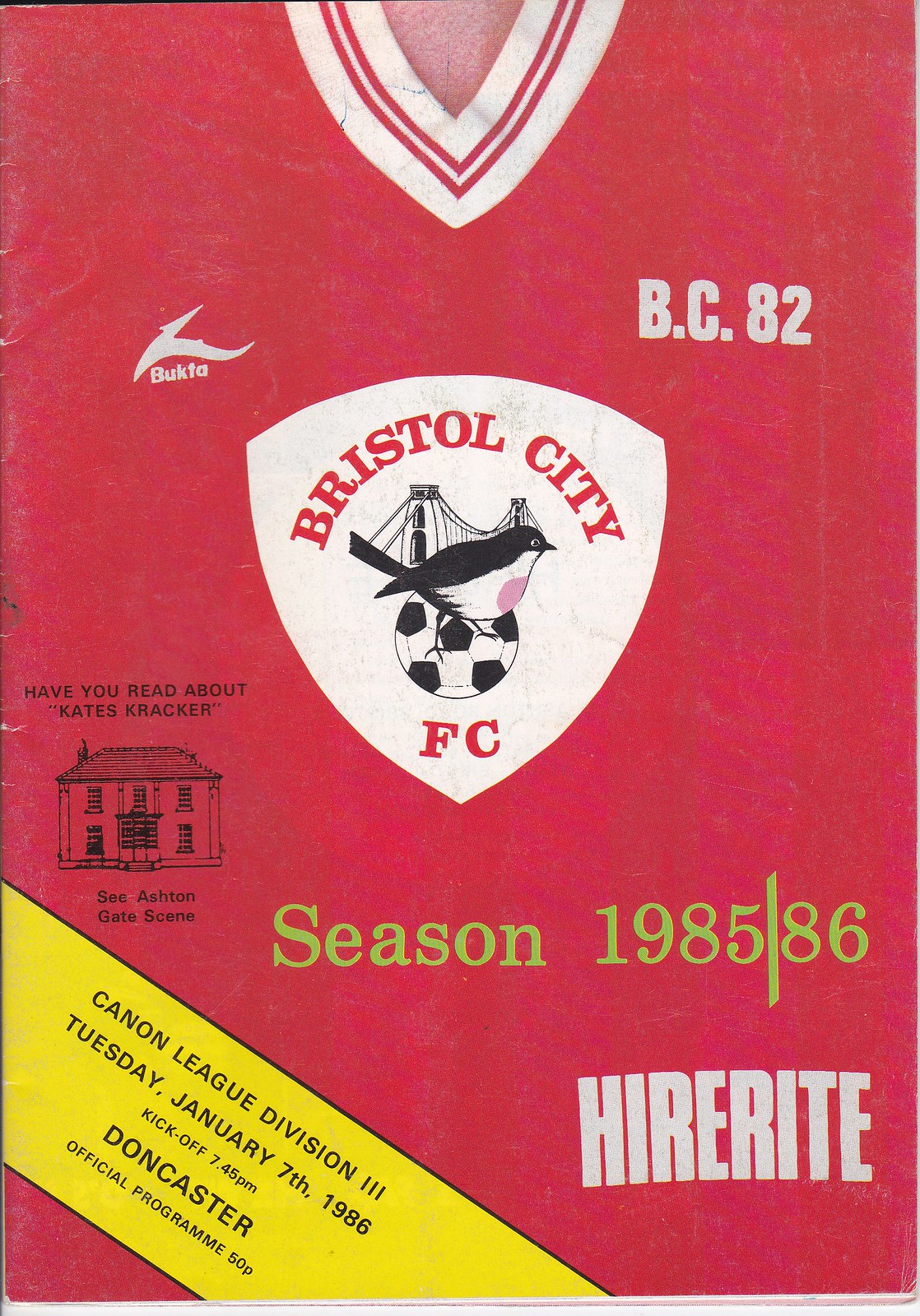The image depicts the cover of a sports program, styled to resemble a team uniform. The dominant background color is red, featuring the neckline of a sports jersey at the top middle, which is white with red stripes. On the upper left, the word "Bukta" is inscribed, and on the upper right, the text "BC82" appears.

Central to the design is a three-sided white shield that contains the text "Bristol City FC" in red letters. Inside the shield, there is an illustration of a bridge, a soccer ball, and a black and white bird nestled between "Bristol City" and "FC." Just below the shield, there is text reading, "Have you read about Kate's cracker? That's the Ashton Gate scene."

Towards the bottom right of the program, yellow text reads, "season 1985 to 86," and below it in white, "HIRE RITE." In the bottom left corner, a yellow strip with black writing displays, "Cannon League Division III, Tuesday, January 7, 1986, kickoff, 7:45 PM, Doncaster Official Program, 50P."